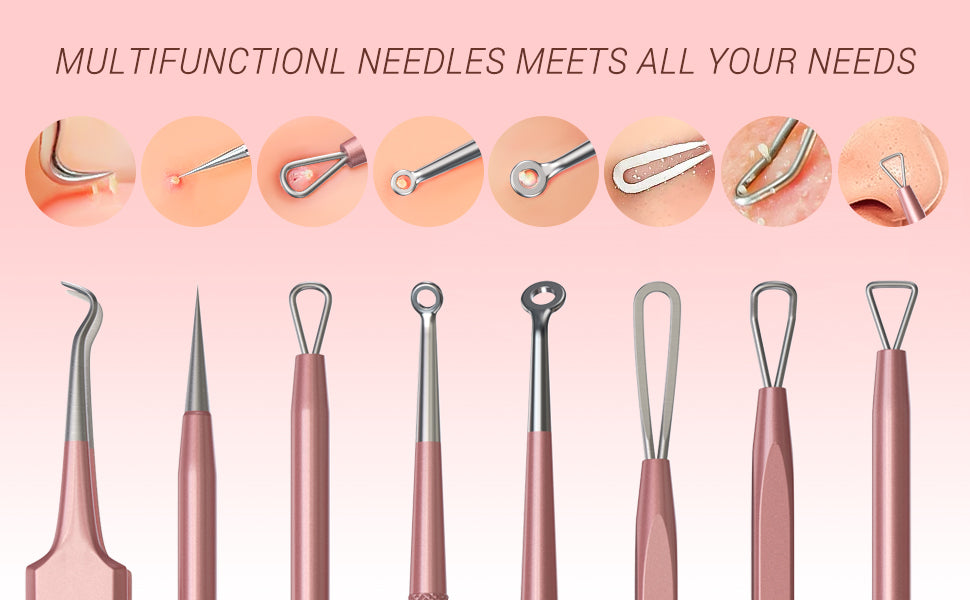The image features a vibrant pink background with the bold phrase "Multifunctional Needles Meets All Your Needs" written in brown lettering at the top. Below the text, there are eight close-up images of various skin issues arranged in a horizontal line, each corresponding to a specific tool. At the bottom, the image displays eight distinct dermatological instruments, each with a pink handle and a metallic tip. The tools include a range of designs: a pointy, curved instrument similar to a dental pick, a straight, sharp needle, and several with different sizes of loops at the ends, all designed to address different skin needs. The consistency in the design hints that these tools are likely marketed towards dermatologists for precise and varied skin treatments.